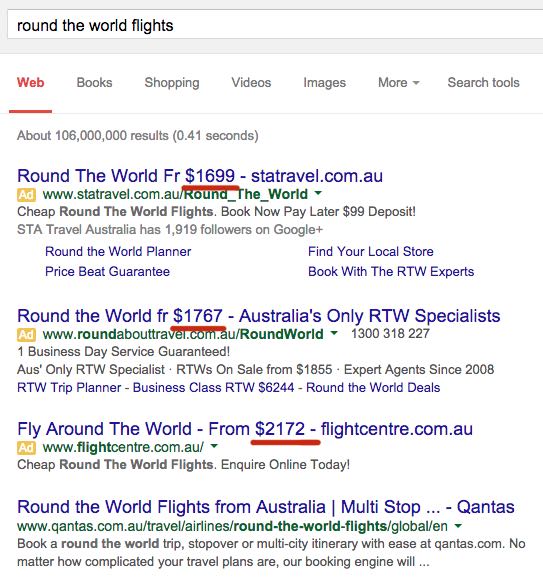This image is a screenshot of a Google search results page. In the Google search bar, the query "round the world flights" is typed in black text. Below the search bar, there are various navigation tabs highlighted in red, including "Web," while other tabs like "Books," "Shopping," "Videos," "Images," "More," and "Search tools" are listed beside it. The results page indicates there are approximately 106 million results found in 0.41 seconds. 

The top three results displayed are sponsored advertisements. The fourth listing is an organic search result for "Round the World Flights from Australia - Multi-Stop Qantas." The website for this result is Qantas.com.au, and it offers options to book a round-the-world trip, including stopovers or multi-city itineraries with ease. The description emphasizes the flexibility of Qantas' booking engine to accommodate complex travel plans. 

The three sponsored ads preceding the organic result are from Australian travel sites, including STA Travel, Round About Travel, and Flight Centre, denoted by their ".com.au" domain endings.